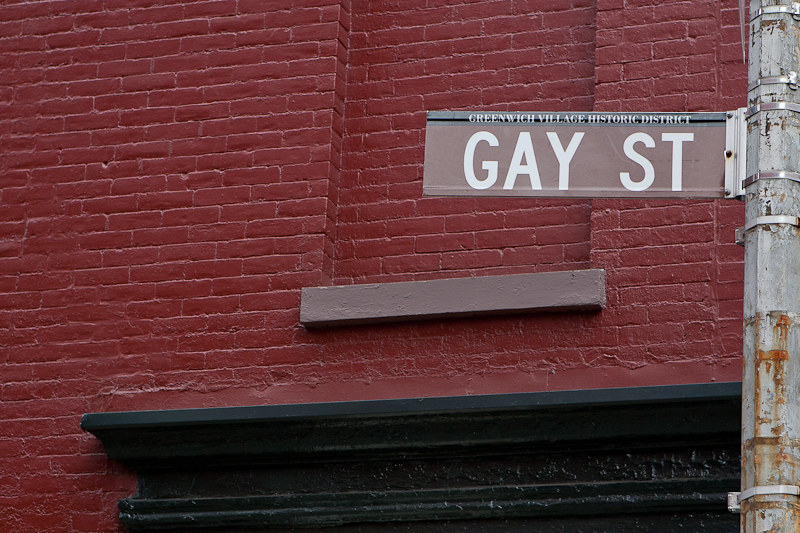This photograph, taken on an overcast day, captures a historic street scene in Greenwich Village. Dominating the image is a weathered silver pole, rusting from years of exposure, supporting a street sign. The sign, painted in a distinct brown color with white letters, proudly declares "Gay Street," with "Greenwich Village Historic District" inscribed in smaller letters above. 

In the background stands an old red brick building, completely painted over in red hues. The building features a black-painted doorway topped with a black awning or molding, suggesting it might house a business. Notably, there is a windowsill painted in slate gray, hinting at a bricked-up window that seamlessly blends into the building's facade. Metal clamps, affirming the sign's steadfast endurance through time, around the pole. The angle of the photograph directs the viewer's gaze upward, adding a sense of grandeur and capturing the historic charm of this iconic location.